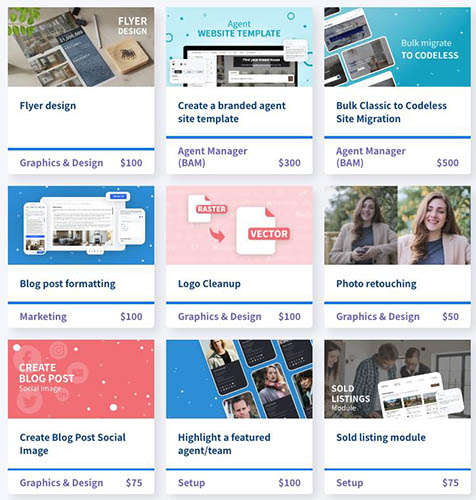This image depicts a well-organized page that showcases a variety of services in a grid layout, structured to provide clear and concise information. The grid is composed of nine distinct services, arranged in three rows, each containing three columns. Each service entry includes a visual representation of the service, followed by the service name, a blue separating line, and the corresponding category or further details.

In the top left corner, there is an entry for a 'Flyer Design.' The visual appears to be an example flyer. Below this image is the text "Flyer Design," followed by a blue line. Underneath the line, the category is labeled as "Graphics and Design," with a price tag of $100 displayed in purple text.

Adjacent to the 'Flyer Design' entry, the next service is 'Agent Website Template.' The image here represents a website template. Below the visual, the text reads "Agent Website Template," followed by a blue line. Underneath this line, the description elaborates with "Create a Branded Agent Site Template," categorizing the service under "Agent Manager."

This page layout, designed for clarity, aims to provide users with a straightforward understanding of the services offered, complete with visual examples, names, descriptions, and pricing where applicable.